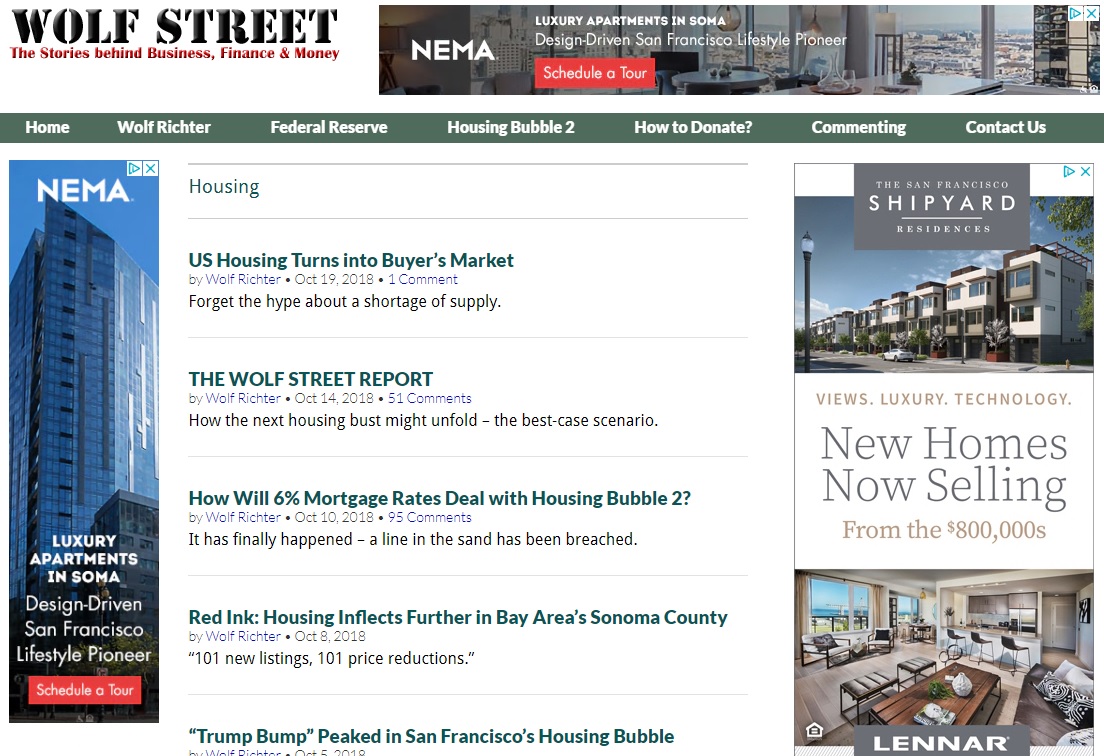The image is of the Wolfe Street website. At the top left corner, the site's title, "Wolfe Street," is prominently displayed in black font. Beneath the title, a subheader reads, "The stories behind business, finance, and money." On the top right, there's a banner that resembles an advertisement. This banner promotes NEMA, featuring the text, "Luxury Apartments in Soma, Design Driven San Francisco Lifestyle Pioneer."

Directly below the banner is the website's navigation menu, which is situated in a horizontal green bar with white font. The menu items, listed from left to right, include: "Home," "Wolfe Richter," "Federal Reserve," "Housing Bubble 2," "How to Donate," "Commenting," and "Contact Us."

On the left-hand side of the page, there's a vertical advertisement for Luxury Apartments in Soma. Correspondingly, on the right-hand side, there are additional vertical ads promoting the San Francisco Shipyard Residences, with a note indicating, "New homes now selling from $800,000."